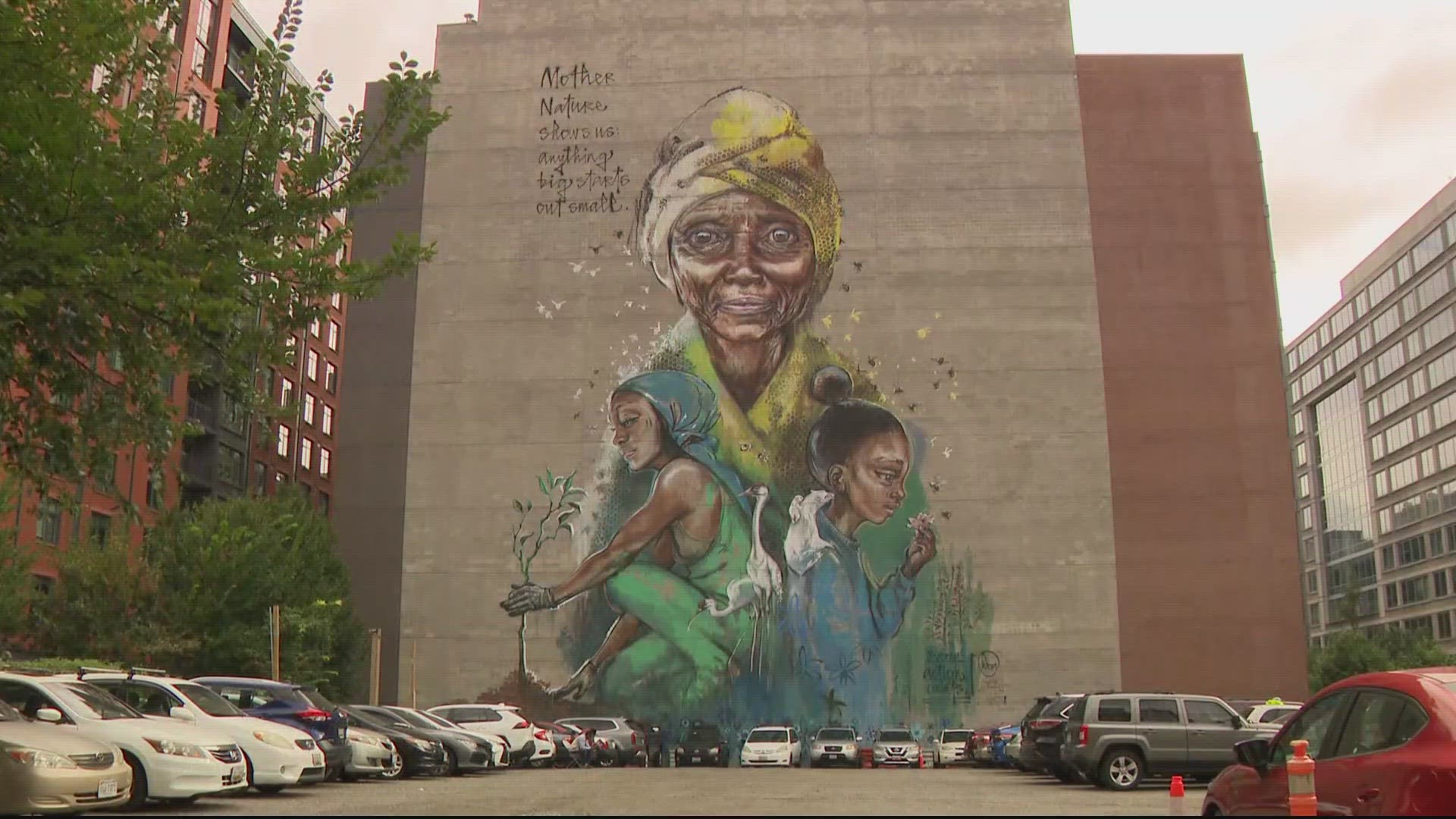This photograph captures an outdoor scene in the center of a parking lot, framed by multi-story buildings with an overcast sky overhead. The parking lot is flanked by rows of cars on both the left and right. Prominently featured is a tall building with a striking mural that spans several stories. The mural showcases three African American females. At the top of the mural, an elderly woman with a head wrap gazes downward. Below her to the left, a woman dressed in green plants a small tree; while to the right, a young girl, with a rodent perched on her shoulder, picks and sniffs a tiny flower. Surrounding these figures are flowers and bees in flight, adding a dynamic element to the scene. Above the mural, in dark script, the words "Mother Nature shows us anything big starts out small" are inscribed. Although slightly blurred, the artist's signature can be found in the lower right corner of the mural. The color palette and imagery of the mural evoke a sense of growth and natural beauty amidst the urban environment.